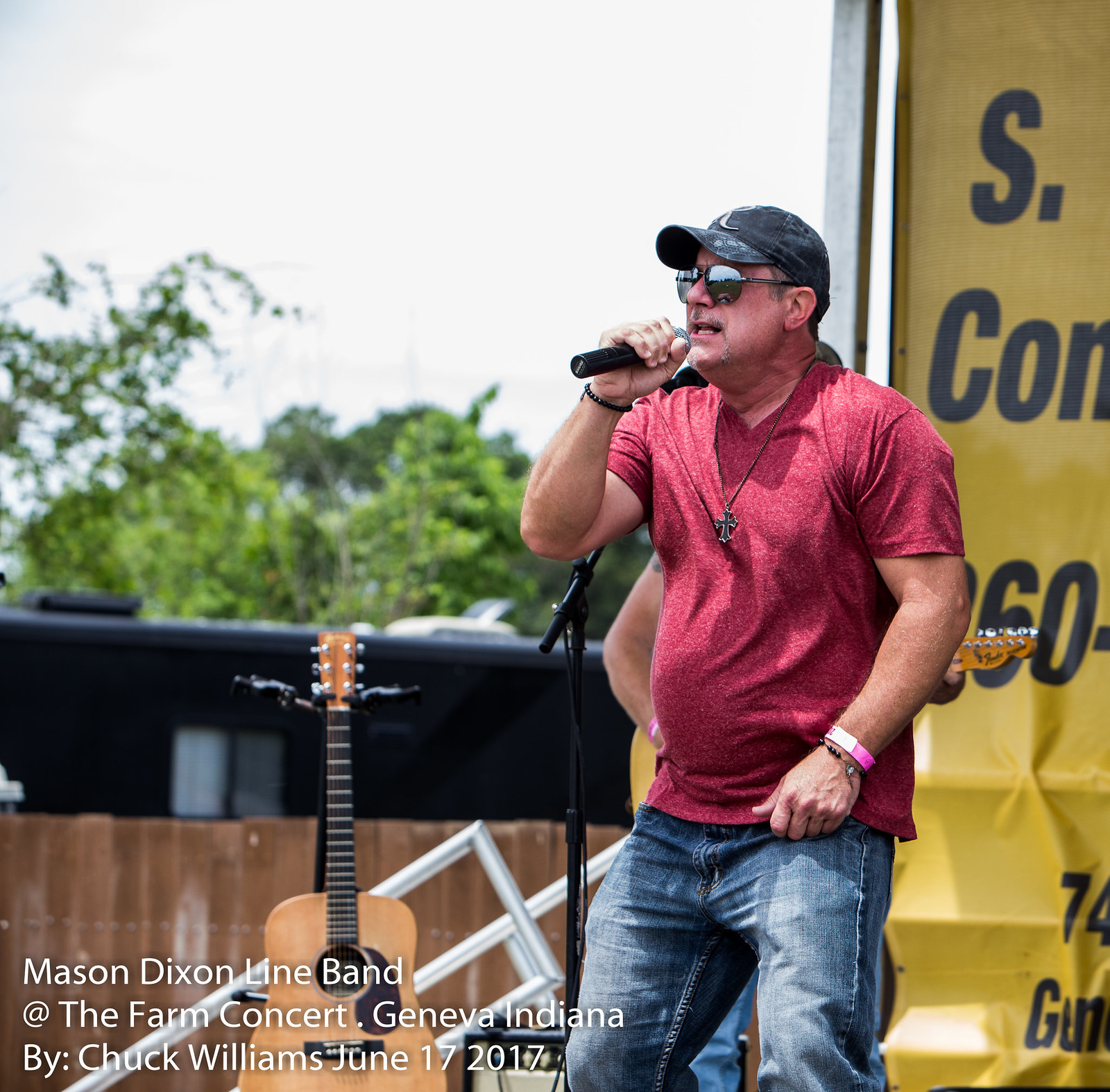The image captures a square format, color photograph of a live performance. Center stage is a white male, apparently either speaking or singing into a black-handled microphone held close to his mouth. He is sporting a heathered red v-neck t-shirt, blue jeans, and a black or blue baseball cap adorned with an unspecified image. His accessories include black aviator sunglasses, a necklace, and a pink and white bracelet on his left wrist. The man has thin gray facial hair.

In the backdrop, a slightly blurred outdoor setting reveals a sky with green tree leaves, suggesting an open-air performance. On the right side of the stage, a yellow banner with visible raised wrinkles hangs, displaying partially cut-off black text starting with "S" and "C-O-M," followed by an unreadable number. Additionally, a dark low building is present in the scene. 

At the base of a brown picket fence to the left of the performer, an acoustic guitar is positioned upright in a stand. Another microphone and a partially visible person playing an instrument can also be seen in the background. In the lower left corner, white text indicates the event details: "Mason Dixon Line Band at the Farm Concert, Geneva, Indiana by Chuck Williams, June 17, 2017." The style of the photograph is described as photographic representationalism realism.